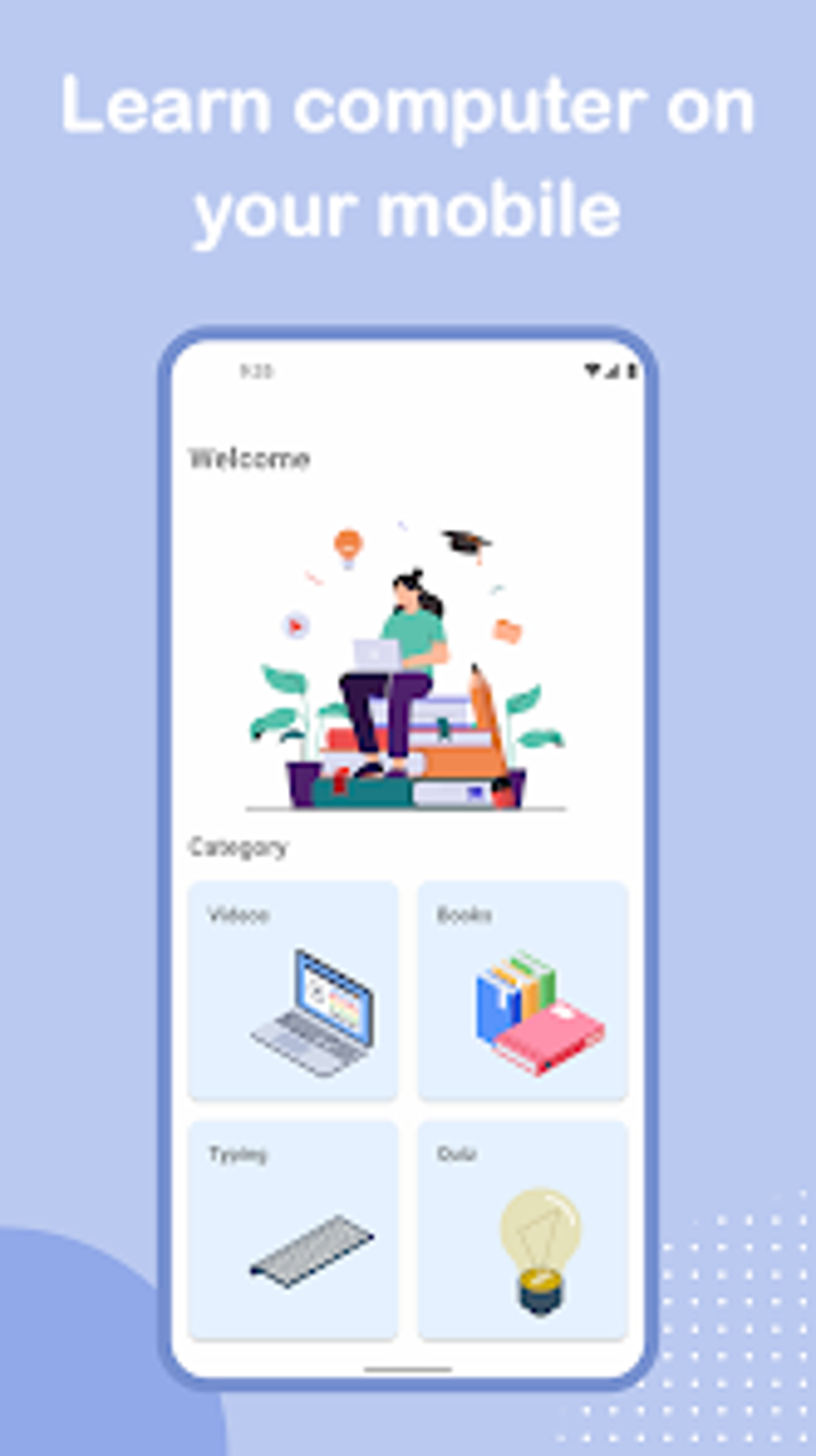The image displays a visually engaging poster set against a blue background. At the top of the poster, crisp white text reads, "Learn Computer on Your Mobile." Below this, a prominent image of a mobile phone fills most of the screen. On the phone’s display, there is a picture of a girl sitting on a bench, working on a laptop. Above her, floating ideas are depicted, symbolizing brainstorming or creativity. Directly above the girl, the word "Welcome" is clearly visible, followed by the word "Category" beneath her.

The image also showcases four distinct rectangular sections, each housing an icon and corresponding word. The first rectangle contains an icon of a laptop labeled "Videos." The second rectangle features an array of colorful books (blue, yellow, green, and red), labeled "Books." The third rectangle shows a keyboard with the label "Typing." The fourth and final rectangle has an icon of a light bulb, although the accompanying text is unclear due to blurriness and poor resolution.